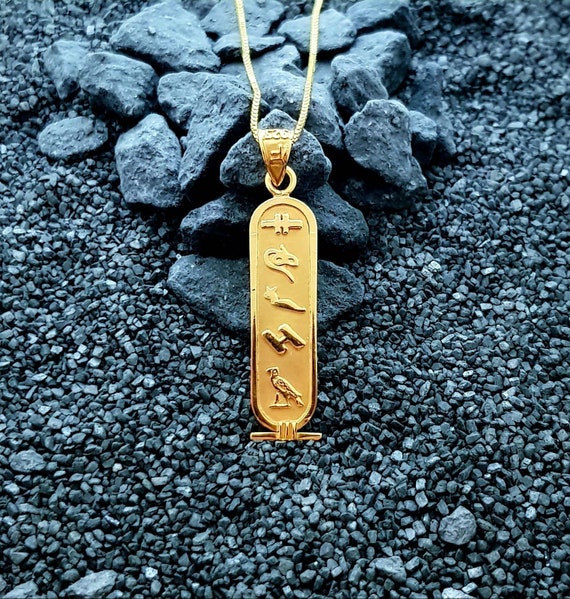The photograph depicts a gold necklace resting on a backdrop of dark, charcoal-colored gravel, overlaid by larger, bluish-gray rocks that mirror the outdoor setting's rugged terrain. The necklace features a delicate, braided gold chain that drapes across the larger rocks, with an oblong pendant hanging over the edge. The pendant, also gold, showcases a series of intricate symbols: a mask representing theater, a bird (likely an owl), a sideways H-like figure, and additional symbols that may be an Egyptian snake or snail, resembling hieroglyphs. The finer details of the pendant, including its golden loop and connecting clasp, harmonize with the overall gold color of the jewelry.